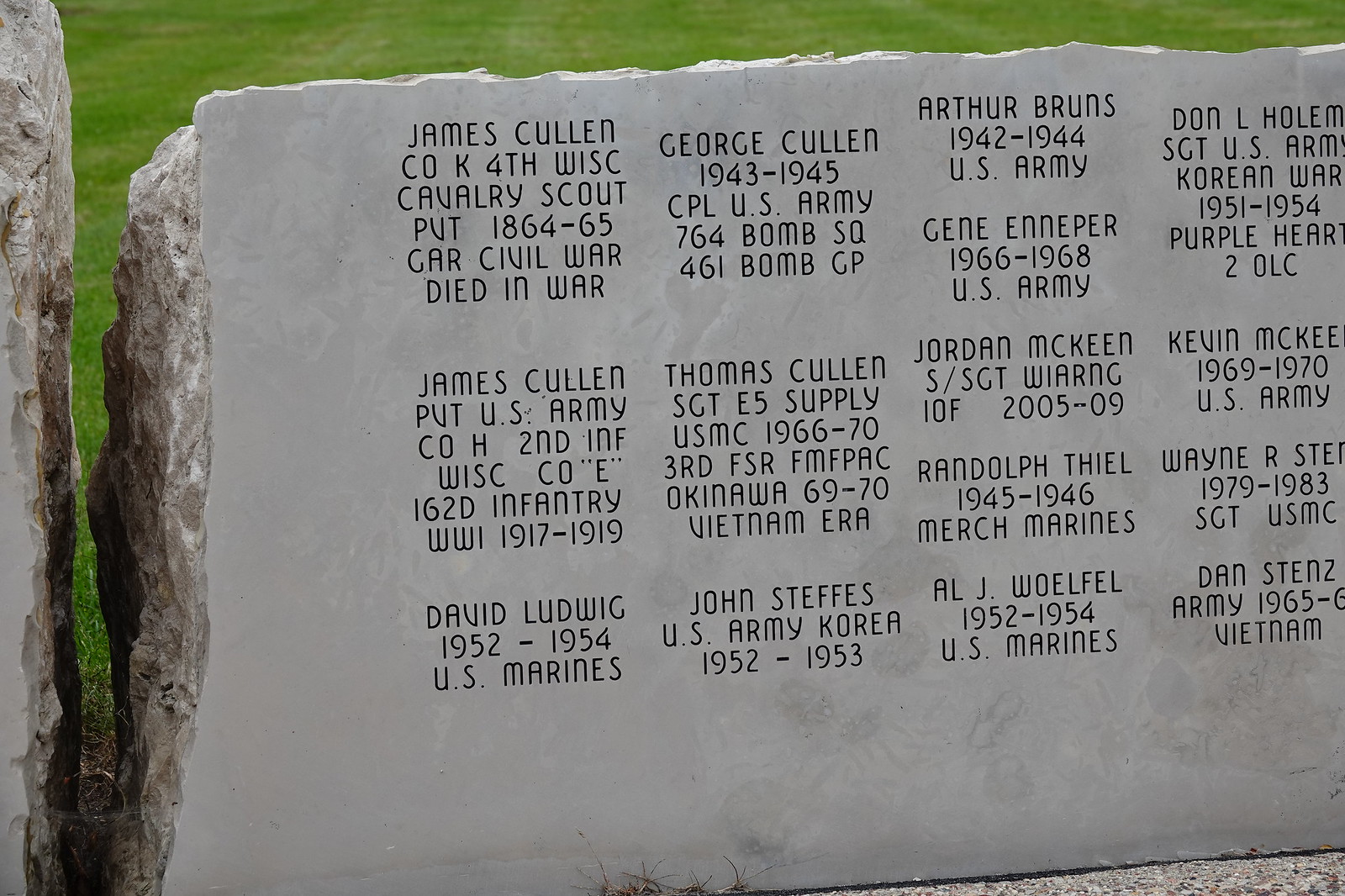The photograph depicts a somber outdoor war memorial set in a neatly trimmed green grassy field. This massive, smooth-surfaced, gray stone monument lists the service details of numerous veterans across three rows and four columns of meticulously etched names. Prominently displayed at the top is James Cullen, C.O.K., 4th Wisconsin Cavalry Scout, who served from 1864-65 during the Civil War and died in service. Beside and beneath his name, you can find others such as George Cullen, Corporal, U.S. Army, 1943-45, Arthur Burns, U.S. Army, 1942-44, and Gene Enneper, U.S. Army, 1966-68. The inscription includes ranks, units, service years, and notable honors such as the Purple Heart, detailing a historical range from the Civil War through the Vietnam era and into the early 1980s. The stone rests upon another slab of stone, with additional names like Don L. Holman, Sergeant, U.S. Army, Korean War, 1951-54, James Cullen of World War I, Thomas Cullen of the Vietnam era, and Randolph Thiel of the Merchant Marines, and extends to the bottom where more veterans like David Ludwig, John Steffes, Al J. Wolfel, and Dan Stentz are commemorated. The grey stone's etched surface contrasts sharply with the visibly rougher side of the rock, suggesting the monument's labor-intense refinement, symbolizing respect and remembrance for the fallen heroes it honors.